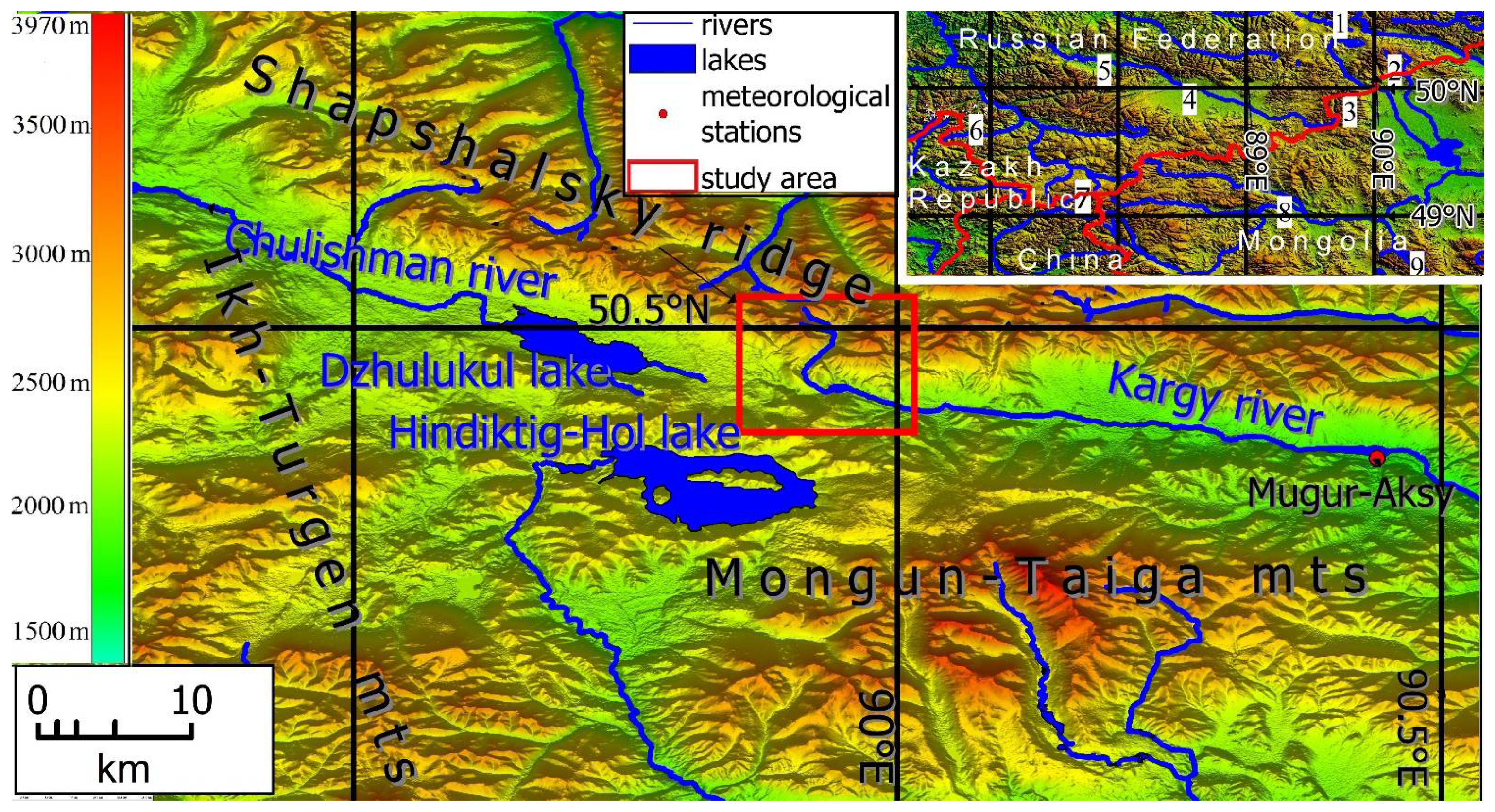This image is a highly detailed, computer-generated topographical map characterized by its crisp lines and bright colors ranging from yellow to green, orange, and red. The map features clear depictions of mountain ranges, valleys, rivers, and lakes, with blue lines indicating waterways. Notably, there is a red square in the center, designating a highlighted study area. Key geographical points include "Shapshalsky Ridge" on the left and "Kargi River" with "Mongoon Taiga MTS" on the right. A legend at the top center of the image explains the symbols: thin blue lines for rivers, blue rectangles for lakes, red dots for meteorological stations, and a red-bordered, white-clear center indicating the study area. Elevations range from 1,500 meters in light blue to 3,970 meters in bright red as illustrated by a gradient scale on the left. A scale bar at the bottom suggests distances from zero to ten kilometers. Additionally, there is an inset map in the top right corner showing a zoomed-out view of the mapped region, which includes labeled areas such as the Russian Federation, Kazakh Republic, China, and Mongolia.